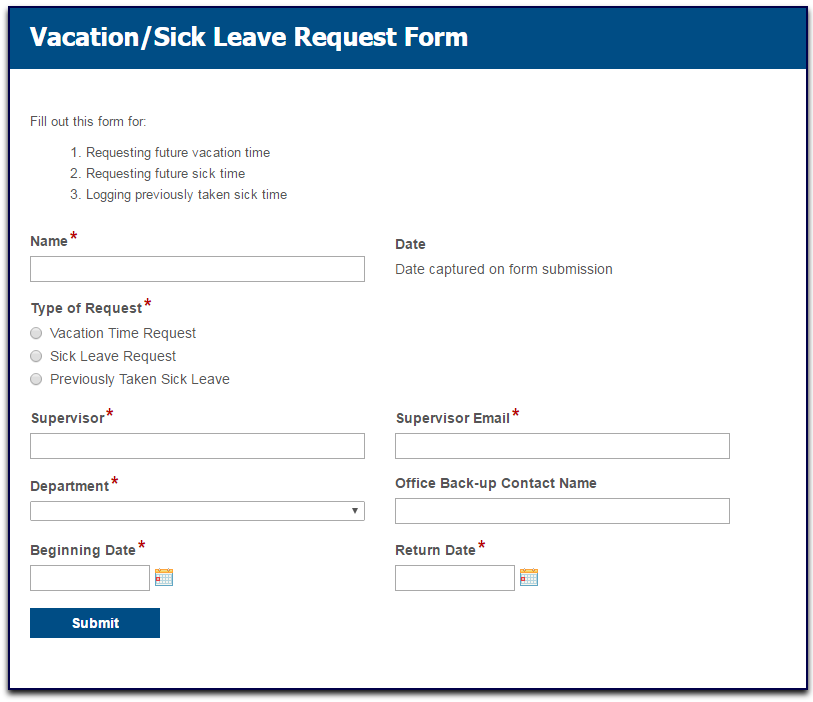**Vacation/Sick Leave Request Form Description**

The form provided is designed for employees to request vacation or sick leave. It features a decorative border and clear sections for user input, ensuring an organized and professional appearance.

- **Borders:** The form is bordered by a thin blue line on the left, right, and bottom sides. The top part of the form features a wider, approximately one-inch blue border.
- **Header:** Within the top blue border, bolded white text reads "Vacation/Sick Leave Request Form," with each initial letter capitalized.
- **Introductory Instruction:** Approximately one inch below the header, in the white section, black text instructs, "Fill out this form for:"
  - **Options:** 
    1. Requesting future vacation time
    2. Requesting future sick time
    3. Logging previously taken sick time

Beneath this instruction, the form is divided into several clearly labeled sections for user input:

- **Personal Information:**
  - **Name:** Bolded with a red asterisk, followed by a long rectangular input field extending halfway across the form.
  - **Date:** On the right side, labeled with "Date captured on submission form" below it.
  
- **Request Type:**
  - Marked bolded with a red asterisk, followed by three gray circles for selection:
    - Vacation time request
    - Sick leave request
    - Previously taken sick leave

- **Supervisory Details:**
  - **Left Side:**
    - **Supervisor:** Labeled with an asterisk, followed by a rectangular input field.
    - **Department:** Labeled with an asterisk, followed by another rectangular input field.
  - **Right Side:**
    - **Supervisor Email:** Labeled with an asterisk, followed by a rectangular input field.
    - **Office Contact Name:** 

- **Leave Details:**
  - **Left Side:**
    - **Beginning Date:** Labeled with an asterisk, with a rectangular input field and a calendar icon on its right.
  - **Right Side:**
    - **Return Date:** Similarly labeled with an asterisk, with a rectangular input field and a calendar icon on its left.

- **Submission:**
  - At the bottom left corner, a blue tab with white lettering reads "Submit."

This detailed layout ensures that all necessary information is captured accurately and efficiently.